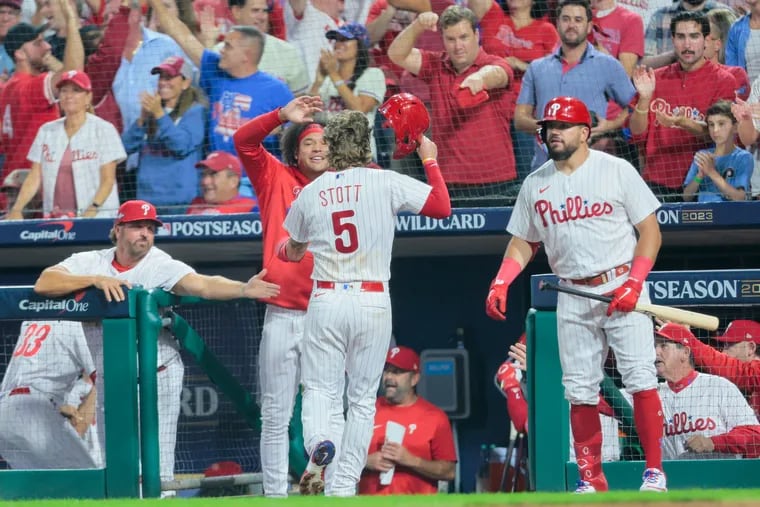In this vibrant image from a Philadelphia Phillies baseball game, Bryson Stott, wearing jersey number 5, is captured running into the dugout, celebrating what appears to be a successful play. Stott is seen holding his red helmet in his right hand, identifiable by the "Stott" and "5" displayed in red on his white uniform. In the dugout, a couple of players are present, sharing in Stott's excitement through high-fives. To Stott’s right is Kyle Schwarber, who is standing on deck with his bat, seemingly about to congratulate Stott as well. Schwarber is donning a red helmet with a white 'P', a white jersey with "Phillies" written in red and blue stars dotting the 'i's, red batting gloves, red socks, and a shin guard, indicating his readiness to bat. The background reveals a lively crowd, most of whom are adorned in Phillies attire, including shirts and hats, and one fan notably wearing a shirt with a Liberty Bell motif. The dugout also features a Capital One advertisement sign marking the game as a postseason wildcard event. The collective excitement suggests that the Phillies have likely just scored, energizing both players and fans in what appears to be a thrilling moment of the game.